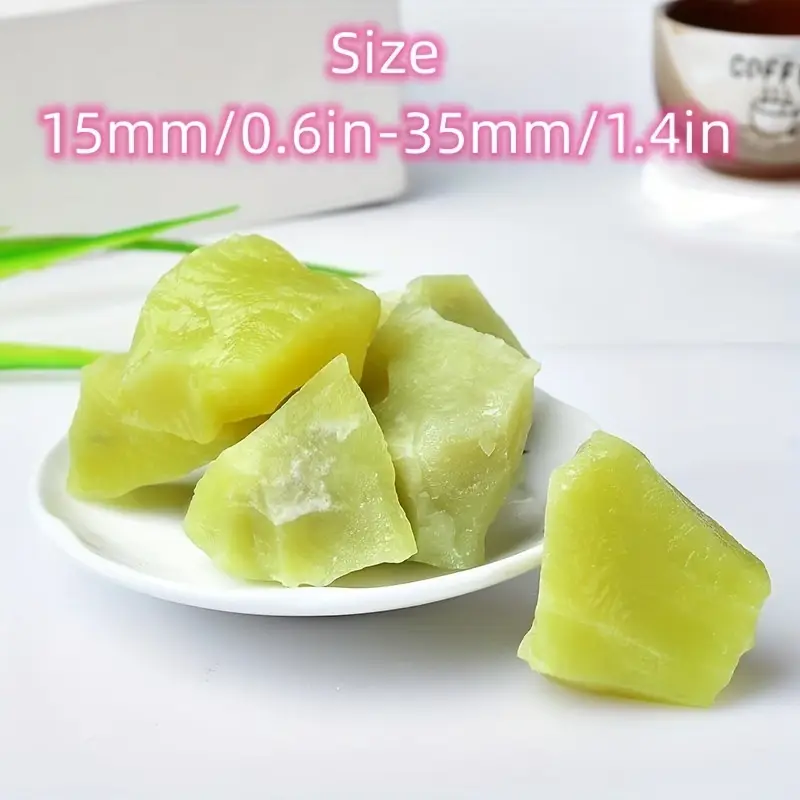The picture showcases a white circular plate placed on a white background, featuring green chunks of an indistinguishable fruit or an exotic food. The green pieces, which have an arresting neon hue, are positioned predominantly on the left side of the plate, and could evoke thoughts of kiwi, melon, or even starfruit, although their exact nature remains uncertain. To the upper right corner of the plate, there is an ivory coffee mug displaying a graphic of a coffee cup and the letters "C-O-F-F," presumably indicating "coffee." Above the main subject, text in white font with a pink outline reads, "Size 15 mm / 0.6 in - 35 mm / 1.4 in," adding specific measurements to the scene. The background suggests an indoor setting, as it's consistent with the white surface the objects rest upon.